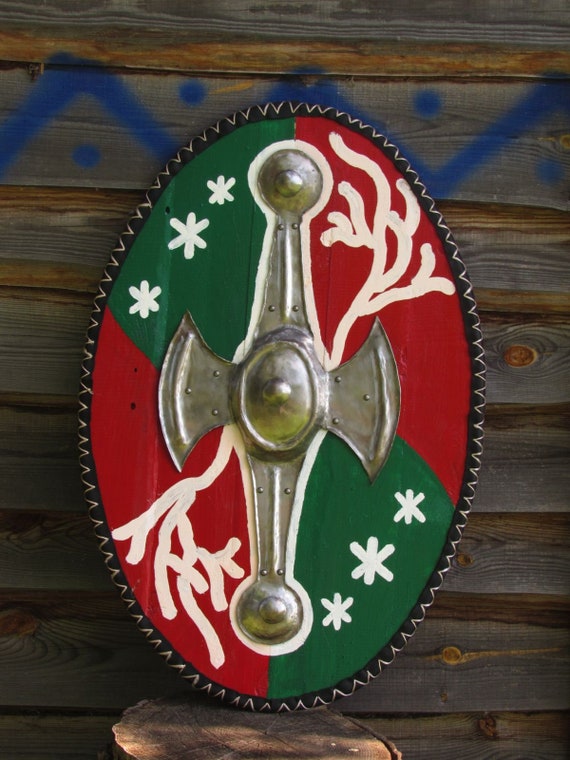This photograph displays a handmade, oval-shaped shield mounted on a dark wooden wall comprised of horizontal planks. The wooden background, which extends from top to bottom in the image, has a distinct blue squiggly line resembling a staircase pattern painted across its top edge. Below the shield, there is a small wooden stump, potentially providing additional support.

At the center of the shield is an intricate metallic design, featuring a central silver circle with extensions resembling axes branching out to the left and right. From the center, an arm extends vertically both upwards and downwards, terminating in rounded tips.

The shield itself is divided into four quadrants with rich hues of green and red. The upper left and lower right sections are green, each adorned with white snowflake-like asterisks. Conversely, the upper right and lower left sections are red, each decorated with white branching lines that resemble tree branches or trunks. Surrounding the shield is a black border punctuated with small brown triangles, giving it a stitched appearance.

The combination of detailed metalwork and vibrant color patterns against the rustic wooden background creates a striking visual contrast, adding to the shield’s handcrafted charm.